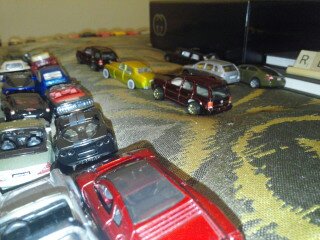This photograph captures an intricate scene of toy cars meticulously arranged on what appears to be a soft, dark gray surface with an olive outline design. Predominantly occupying the left side of the image, there are two lines of toy cars parked extremely close together, with approximately five cars in each row butted up against each other. The toy cars here showcase a variety of colors, with a red car and a silver car being the most prominent in the foreground.

Adjacent to these rows is another closely packed line of three toy cars arranged front to back. This line includes a black car, a goldish-green car in the center, and a larger dark brown van at the end. To the right of this row are three more cars, spaced slightly apart: a gray car, an avocado green car, and another black car.

In the background, the surface appears to be strewn with sand across the gray asphalt-like material. A gray sky creates a somber horizon where more toy cars are faintly suggested. A large black structure at the back of the picture also includes visible letters from a Scrabble tile, specifically the letter 'R', adding to the playful yet enigmatic nature of the scene. The upper right-hand corner of the image features a shiny black object, possibly a book or a large block, further adding depth and intrigue to the composition.